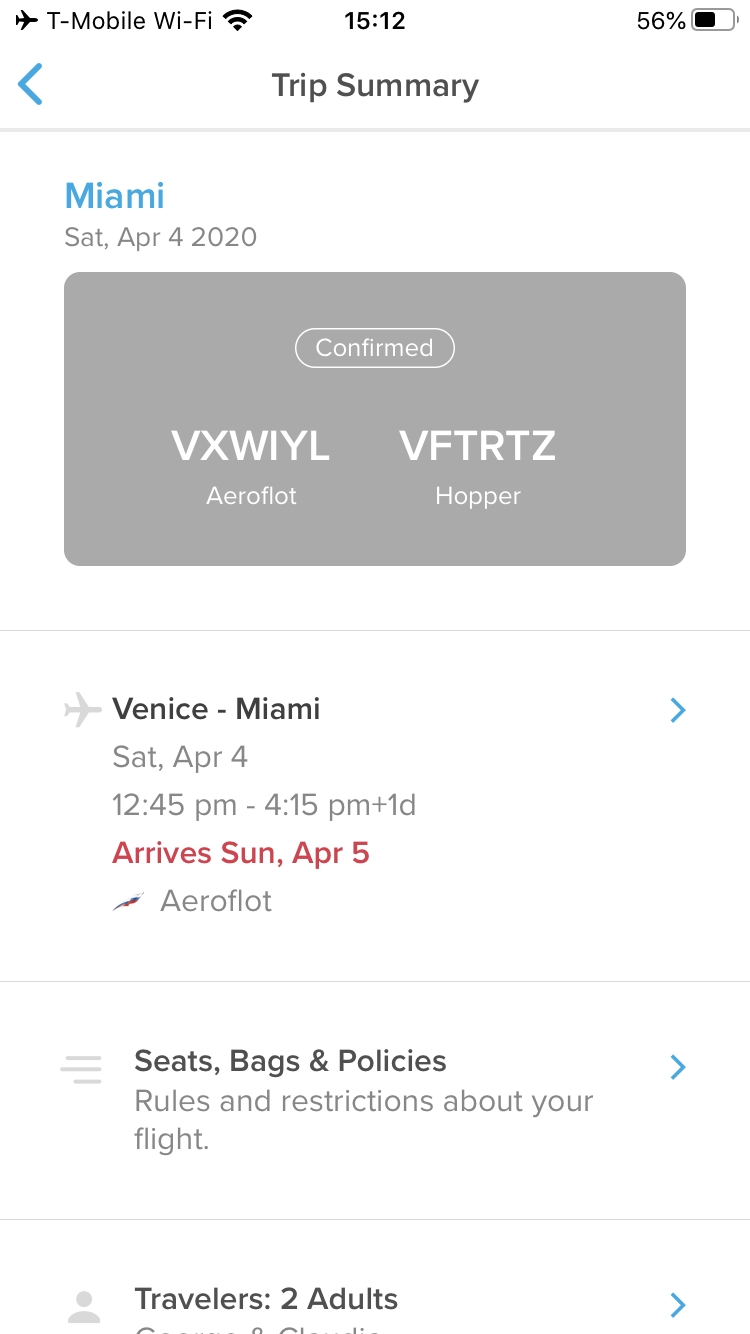This is a detailed caption for the image:

---

Screenshot of a flight itinerary captured on a T-Mobile mobile device. The document is titled "Trip Summary" and outlines travel details for a journey to Miami on Saturday, April 4th, 2020. The flight is confirmed with Aeroflot, facilitated by Hopper. While the full itinerary is partially cut off, the visible details indicate a first leg from Venus to Miami. Below this segment, options to view seats, baggage policies, and other travel policies are available. The screenshot also indicates that two adults are traveling, although the remaining information is obscured.